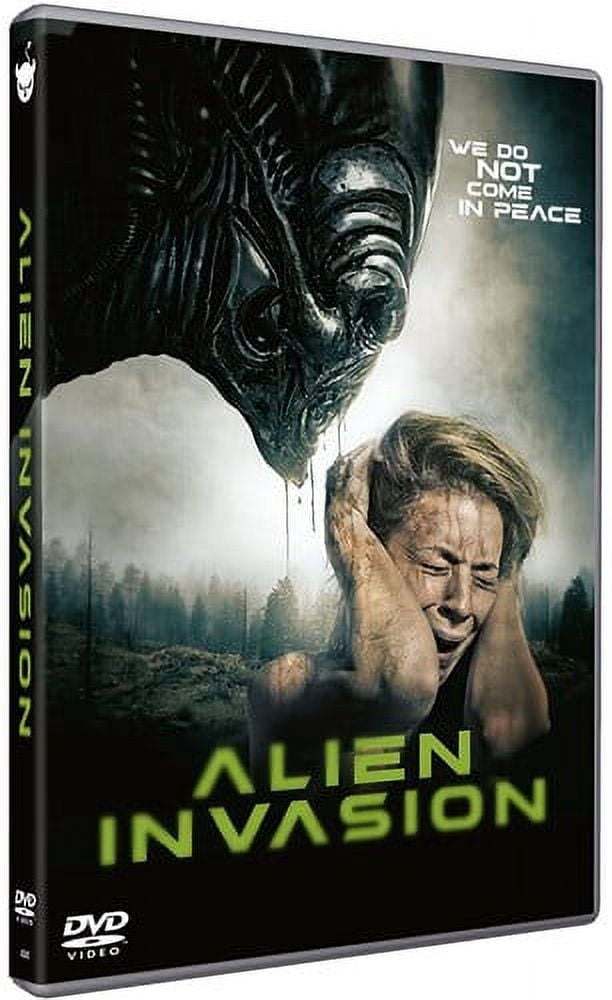This image is a detailed depiction of a DVD cover for a B-grade sci-fi movie titled "Alien Invasion." The background of the cover is predominantly white, with striking elements drawing attention to the alien-themed content. On the front of the cover, the upper section prominently features the menacing face of a black alien, reminiscent of the creature from the classic "Alien" movie. Below the alien, a terrified blonde woman, presumably trying to escape, covers her ears in fear. The background portrays a surreal forest setting with rocky terrain and a sky filled with white clouds.

The title "Alien Invasion" is boldly printed in light green at the bottom of the cover. The tagline "We do not come in peace" is visible in white at the top right corner, adding to the ominous atmosphere of the image. The bottom left corner displays the "DVD video" mark, indicating the format.

Additionally, the image provides a side view of the DVD cover, revealing a black spine with the title "Alien Invasion" in green and a small white devil logo at the top. The same "DVD video" label appears at the bottom of the spine. This comprehensive view gives the impression of someone inspecting the DVD case from different angles, emphasizing the distinct elements and overall theme of the film.